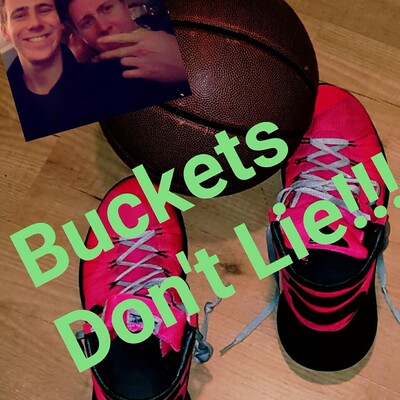This detailed image depicts a carefully arranged collage of photos, creating a dynamic and vibrant scene. Dominated by a pair of striking black and red high-top sneakers with gray laces, the centerpiece of the collage features these shoes viewed from an overhead angle, resting next to an old, worn brown basketball. The basketball, placed between the sneakers, adds a nostalgic touch to the arrangement. 

In the top left-hand corner, there is a small photograph of two men, likely in their twenties, posing together. One of the men is making a peace symbol with two fingers in front of his mouth. Their photo, though small, is a significant part of the composition as it adds a personal and human element to the otherwise object-focused image. 

Spanning diagonally from the lower left to the upper right across the middle of the collage, the phrase "Buckets Don't Lie!!!" is prominently displayed in a bright lime-green font, adding a bold and energetic text element to the visual. This message, coupled with the imagery of basketball and sneakers, hints at themes of sportsmanship and athletic lifestyle. The entire composition is set in a vertical, square frame, enhancing the collage's compact and dynamic feel.